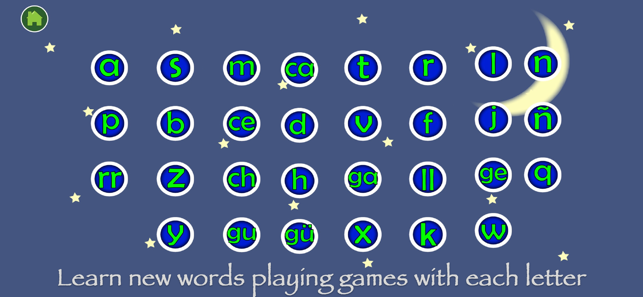The image features a light blue background adorned with scattered white stars, creating a whimsical and inviting night sky theme. Nestled in the top right corner is a white crescent moon, adding a touch of celestial charm to the scene.

At the bottom of the image, the caption "Learn new words playing games with each letter" is prominently displayed, encouraging an educational and playful experience.

Across the middle of the image are rows of dark blue circles, each encircled by a white border. Inside each circle is a lowercase letter in vibrant green, standing out clearly against the blue background.

In the top row of circles, the letters A, S, M, C, A, T, R, L, and N are arranged from left to right. The second row features the letters P, B, C, E, D, V, F, J, and N. Further down, the third row displays letters R, R, Z, C, H, H, G, A, L, L, G, E, and Q. Finally, the bottom row contains the letters Y, G, U, Ü (U with two dots over it), X, K, and W. This strategic arrangement of letters hints at an educational game designed to help users discover and learn new words through engaging and playful interaction.